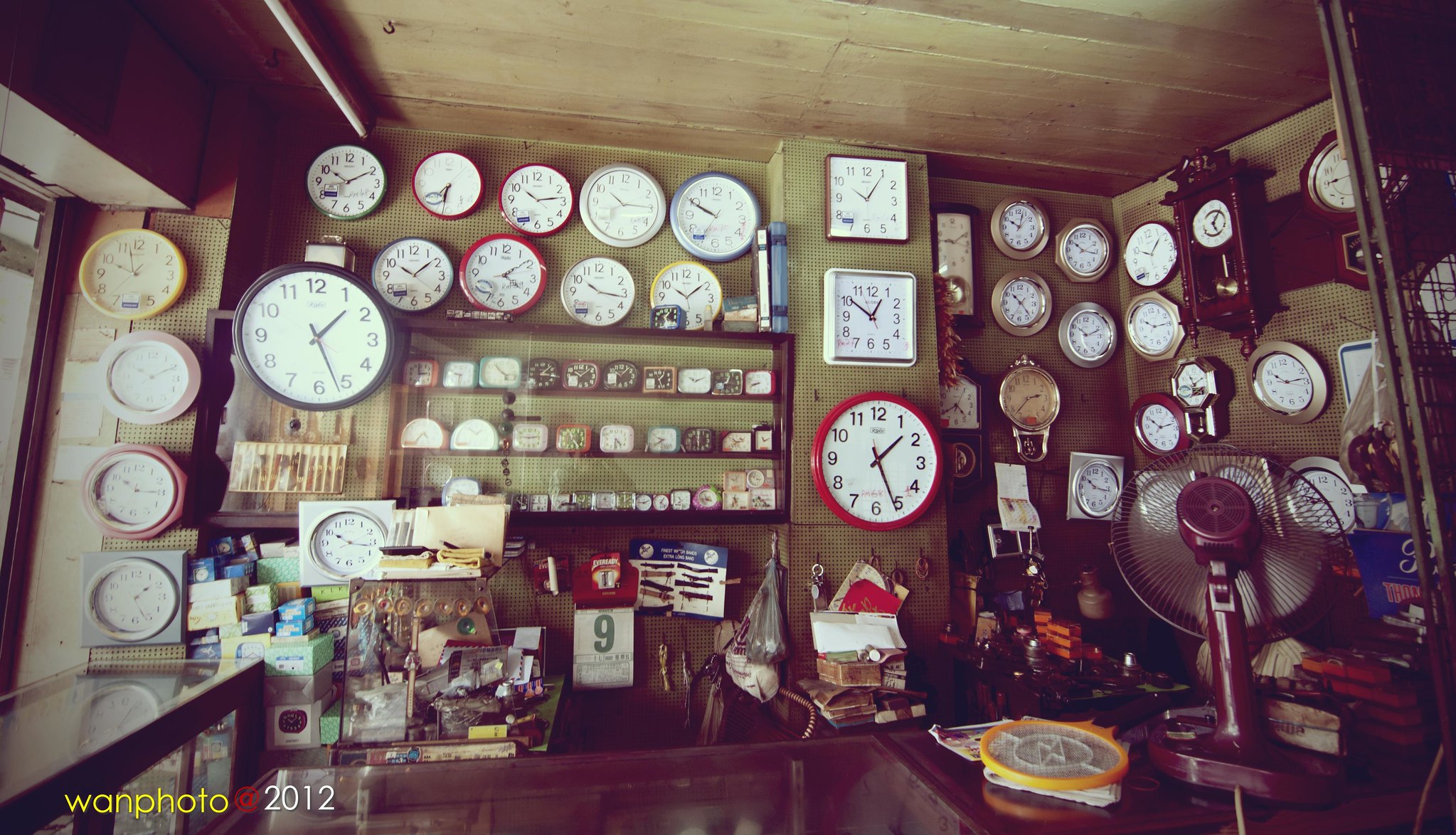The photograph depicts the interior of a vintage clock store filled with a myriad of clocks. The walls are adorned with an extensive assortment of timepieces in varied shapes, sizes, and colors. On the right-hand side, a quaint mini grandfather clock stands out among the collection. Dominating the room, clocks with white faces and bodies in hues of yellow, pink, brown, silver, and more are visible. Central to the image are two white square clocks mounted on a pole, beneath which hangs a round clock framed in red. The top left section features five clocks in a row, followed by four more clocks directly beneath, primarily in white and red. Below these, three additional rows each contain nine smaller clocks.

On the left side, shelves house various colored boxes, likely for storage. There is an olive green case and a dark chocolate brown glass case among the clutter. Light streams in from a large window on the left center part of the room. Noteworthy details include a fan with a maroon red base and cylindrical neck, positioned on a dark chocolate brown countertop. A calendar marked with the number nine can be found around the middle area of the wall.

At the top of the photograph, the ceiling is lined with alternating light and dark brown wooden beams. The olive green wall color complements the eclectic mix of timepieces. The photograph is stamped with the marking "WANPHOTO 2012" in yellow and white font with a small red symbol.